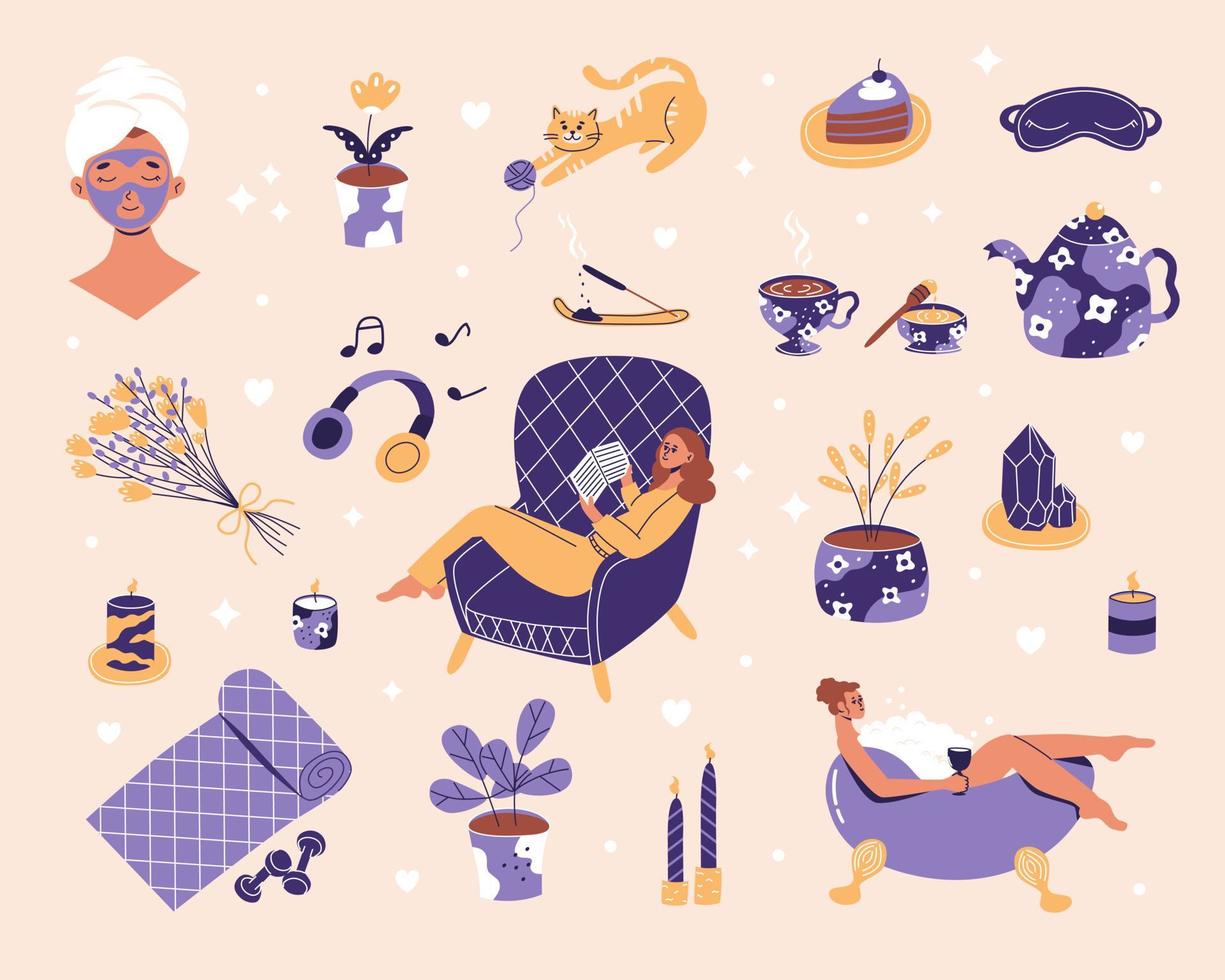The image features a soft, peach-yellow background adorned with a variety of clipart-style illustrations that predominantly incorporate shades of purple alongside other colors, arranged in a loosely structured grid. Key elements of this vibrant composition include:

- **Top Left**: A woman with a purple facial mask and a white towel wrapped around her head, her eyes closed in relaxation.
- **Top Row**: A potted plant with yellow petals and butterfly-wing-shaped leaves in a purple pot with white clouds, a yellow cat playing with a purple yarn ball, a slice of purple cake with white frosting and a purple cherry on a yellow plate, and a purple sleep mask with closed eyes and eyelashes design.
- **Second Row**: A purple teapot decorated with white flowers, a matching cup of honey with a wooden honey dipper, a purple coffee cup with white flowers filled with coffee, a mysterious object resembling the bottom of a dress shoe with a dripping incense stick, purple and yellow headphones, and yellow flowers with small red buds and purple leaves.
- **Center**: A woman with dirty blonde hair in yellow pajamas or a tracksuit, reading a book while seated in a purple chair with yellow feet and white grill marks at the back.
- **Center Right**: A purple geode on a yellow plate, a purple cylindrical candle with yellow wax and flame, a Victorian-style purple bathtub with yellow legs, a woman relaxing inside holding a wine glass, alongside purple candles with white stripes, and another potted plant similar to the teapot's design.
- **Bottom Left**: A half-rolled purple yoga mat with white grill marks, small purple dumbbells beside it, and two types of candles—one a yellow dish with purple swirls and yellow flame, and another smaller purple candle with white flower patterns and orange flame.

The overall visual theme revolves around the contrasting yet harmonious combination of purple and yellow hues in objects ranging from everyday items to whimsical elements, creating a cohesive and playful tableau.